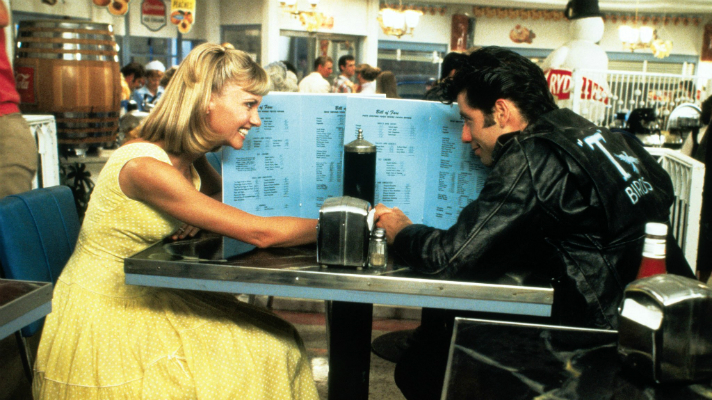The image is a detailed film still from the movie Grease, featuring a scene set in a cozy diner with a classic, metallic-topped table supported by a black pedestal. Sandy, the main character with shoulder-length blonde hair and bangs, sits on the left. She is wearing a sleeveless yellow dress with a white polka-dot pattern and a poofy skirt. Tanned and smiling brightly, she gazes at John Travolta's character, seated across from her on the right. He sports a black leather jacket with the word "T-Birds" and an illustration of a bird on the back, along with slicked-back, greasy black hair and prominent sideburns. Both characters are holding hands, their clasped fingers resting on the table, partially concealed behind an upright menu. Surrounding them on the table are typical diner items, including a container of napkins, salt and pepper shakers, and a straw holder. In the background, the bustling atmosphere of the diner is visible, with workers and other patrons eating. Both Sandy and the man are sharing a moment of intimacy, smiling at each other warmly.